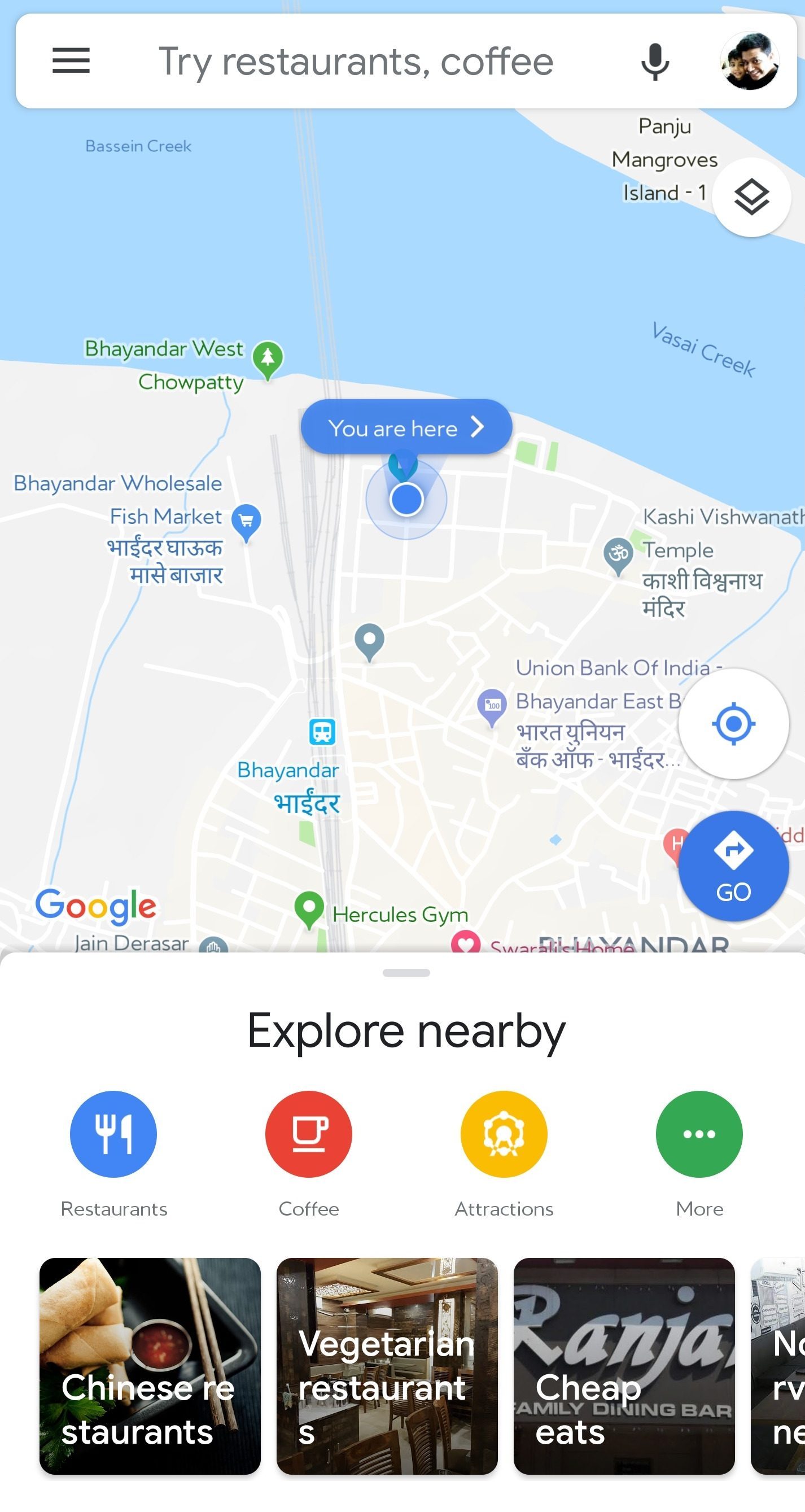This image showcases a detailed view of a Google Maps webpage. Dominating the screen is a large, interactive map, with water bodies illustrated in the upper portion. A light gray line runs diagonally from the top to the side of the map, intersecting the edge. Prominently displayed on a large white banner, the text reads "Try Restaurants, Coffee," accompanied by an icon of a microphone and a profile picture featuring two individuals with brown hair.

Beneath the water, the landmass is depicted in white, with a notable blue dot indicating "You are here" located in the upper section of the map. Scattered throughout, various pins in shades of blue, gray, and green mark locations, highlighting specific spots such as banks and a restaurant.

In the bottom portion of the map, a significant blue circle with the word "Go" displayed inside is visible, with a diamond-shaped arrow pointing to the right. The Google Maps logo, characterized by its blue, red, gold, and green palette, is positioned in the lower left-hand corner of the image.

Directly below the map, a section urges users to "Explore Nearby," embellished with colorful circles labeled "Restaurants," "Coffee," "Attractions," and "More" in Google’s signature hues. Below this, there are rectangular boxes that appear to be advertisements; the first features an image of food with captions such as "Chinese restaurants," "vegetarian restaurant," and "cheap." Additionally, there is a partial image of another food-related advertisement.